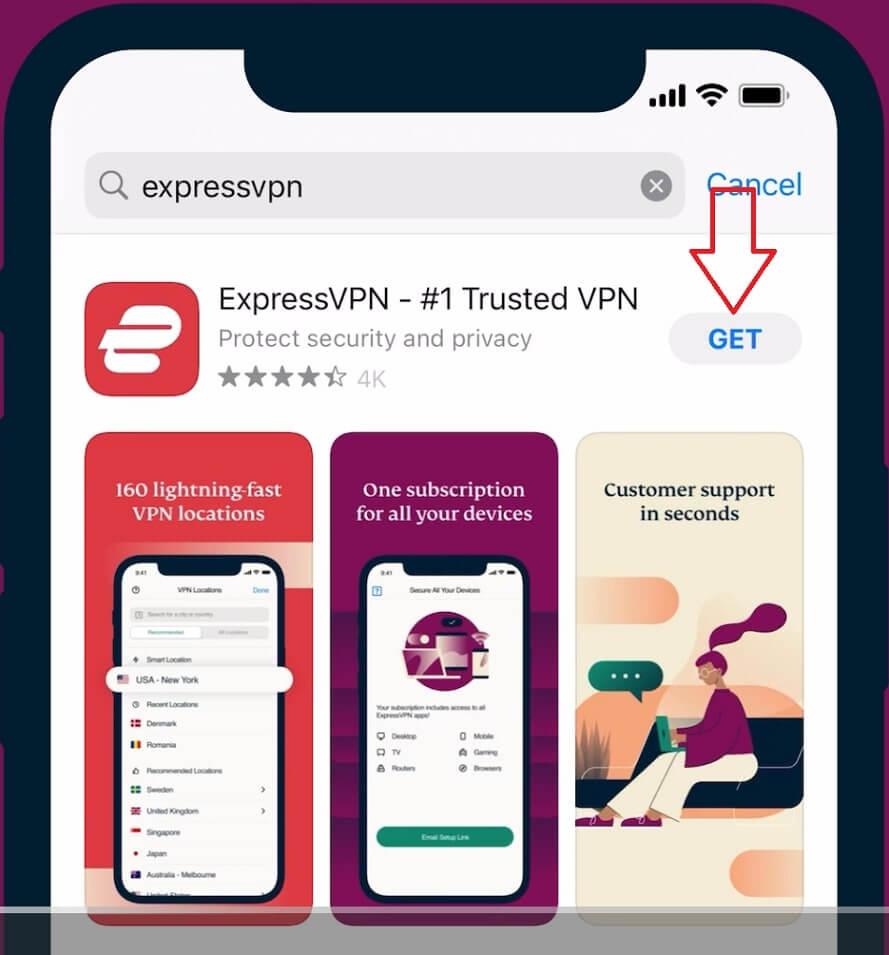This image is a screenshot taken on a mobile phone, displaying the search results from an app store query for "ExpressVPN." At the top of the screen is a search bar where "ExpressVPN" is typed in. Directly below the search bar, there appears the search result for the app "ExpressVPN – #1 Trusted VPN."

The app's logo is prominently featured, showcasing a red square with a stylized white "E" within it. The app has garnered a 4.5-star rating from approximately 4,000 reviews. On the upper right-hand side of the screen, there's a blue button labeled "GET," suggesting that users can click it to download the app.

Adjacent to the app title are three promotional images designed to highlight its features. The first image, which dominates the visual space with a red rectangular background, emphasizes the message "160 Lightning-Fast VPN Locations" and highlights "United States - New York" as one of the available locations.

An arrow icon on the upper right portion of the screen points downwards towards the "GET" button, indicating where users can click to initiate the download of the ExpressVPN app.

In summary, this screenshot serves as a clear guide for users on how to find and download the ExpressVPN app, complete with visual aids and highlighted features.